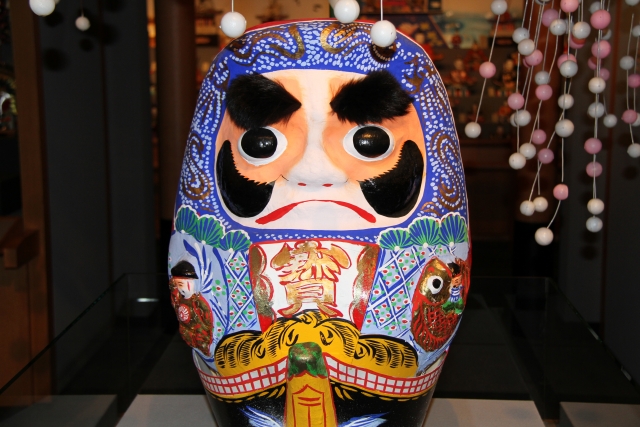The image showcases a vividly colorful centerpiece, capturing what appears to be an egg-shaped figure with a man's face that carries an expression of slight grumpiness. This character, positioned in the middle of the image and seemingly resting on a glass table, is adorned with an array of colors—prominent shades of blue, red, yellow, green, along with highlights of black, white, pink, purple, orange, and tan. His face is distinguished by thick, bushy black eyebrows and black beady eyes, with a frown represented by a single red stripe for a mouth. The mask-like visage features a white stripe running down the center, merging with additional white paint across his mouth, and black cheeks. The figure's head is encased in a colorful covering reminiscent of a balaclava, decorated with intricate designs including images of a man and a fish. The setting suggests a dimly lit restaurant with an Asian theme, enhanced by hanging marbles, pink and white, strung from the upper right side of the frame. The overall ambiance is dark, focusing all attention on the central, elaborately adorned figure.